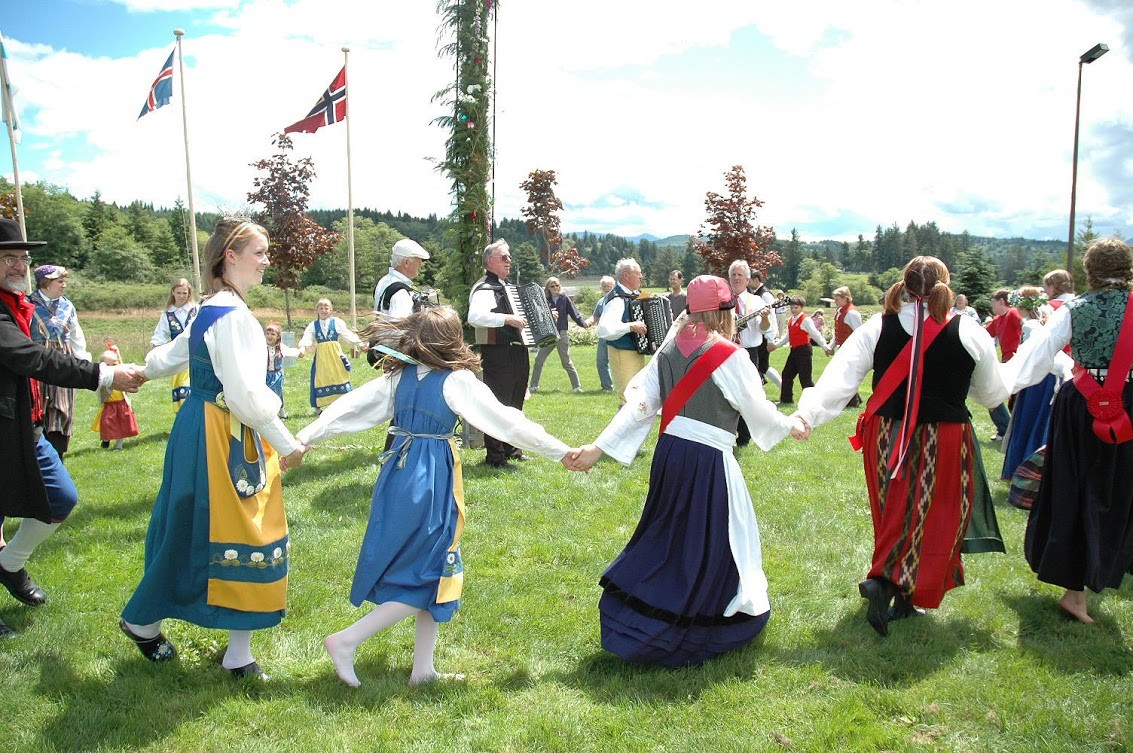The image depicts an ethnic or cultural festival likely of European origin, featuring a lively outdoor scene set in a grassy area with trees in the background. In the forefront, a group of predominantly Caucasian women, dressed in traditional Bavarian-style long dresses with dark colors and white long sleeves, are holding hands and dancing in a circle. Some of the women also wear head coverings. Surrounding them are older men, likely in their 50s or 60s, playing musical instruments such as accordions and a stringed instrument. The men are dressed in traditional outfits as well, with some possibly wearing kilts. A central pole or tree, serving as the focal point of the dance, suggests this could be a spring celebration. Scattered flagpoles with partially visible flags flutter in the background, and the sky above is bright with white clouds, giving a festive yet calm ambiance to the scene.